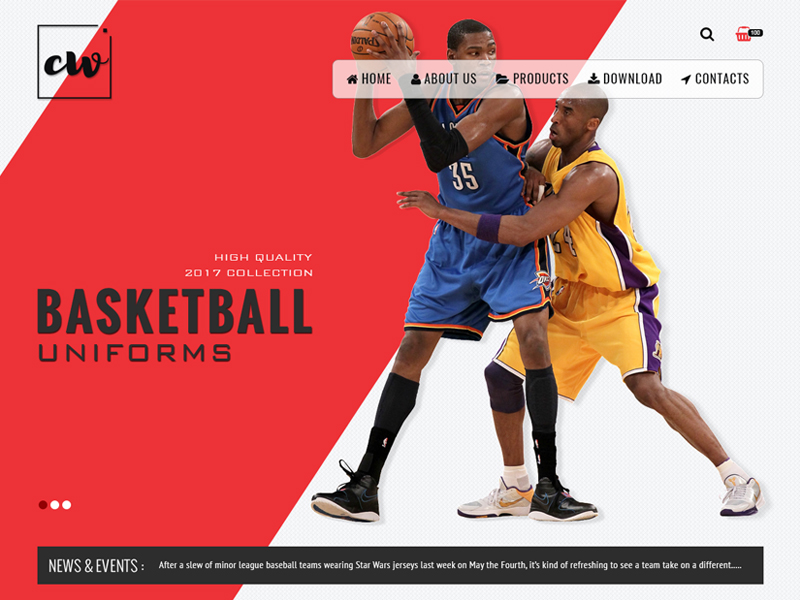The image depicts an intricately designed store interface. The layout starts with a gray border spanning approximately two inches from the left to the right at the top, angling downward for about two inches on the left side. From there, a diagonal red section extends downwards to approximately three inches from the right corner at the top, intersecting with a point about three inches from the left bottom corner before transitioning into a white section below.

In the top left corner of the image, there is a unique square with a missing right corner. Inside this irregular square, a small dot houses a stylized, bolded, black cursive "CW." Centrally located within the red section, the text reads, "High Quality" in small white letters, followed by "2017 Basketball Collection."

On the left side of the red section, bolded in black and entirely capitalized, the word "BASKETBALL" appears above the smaller word "UNIFORMS." Further down within the white section are three dots in a sequence: red, white, and white.

At the bottom of the image, a large black rectangle spans the entire width, overlapping into the white background. Inside this rectangle, the words "News and Events" are prominently displayed. In smaller letters beneath, there’s a brief news excerpt: "After a slew of minor league teams wearing Star Wars jerseys last week on May 4th, it's kind of refreshing to see a team take on a different..."

The central visual feature of the image is a photograph of Kevin Durant. He is pictured with his chest facing forward, holding a basketball at head level. Durant's uniform is blue and orange, complemented by black socks and black shoes with white soles. To his right, Kobe Bryant is depicted guarding him, reaching around Durant's waist. Kobe wears a yellow uniform with purple stripes down the ribcage and the sides of the shorts, along with white and purple shoes and a blue wristband.

Above the players, a white tab runs horizontally from left to right, containing various icons and labels for navigation: a home icon labeled "Home," a profile icon labeled "About Us," a photo icon labeled "Products," a download icon labeled "Download," and a search icon labeled "Contacts."